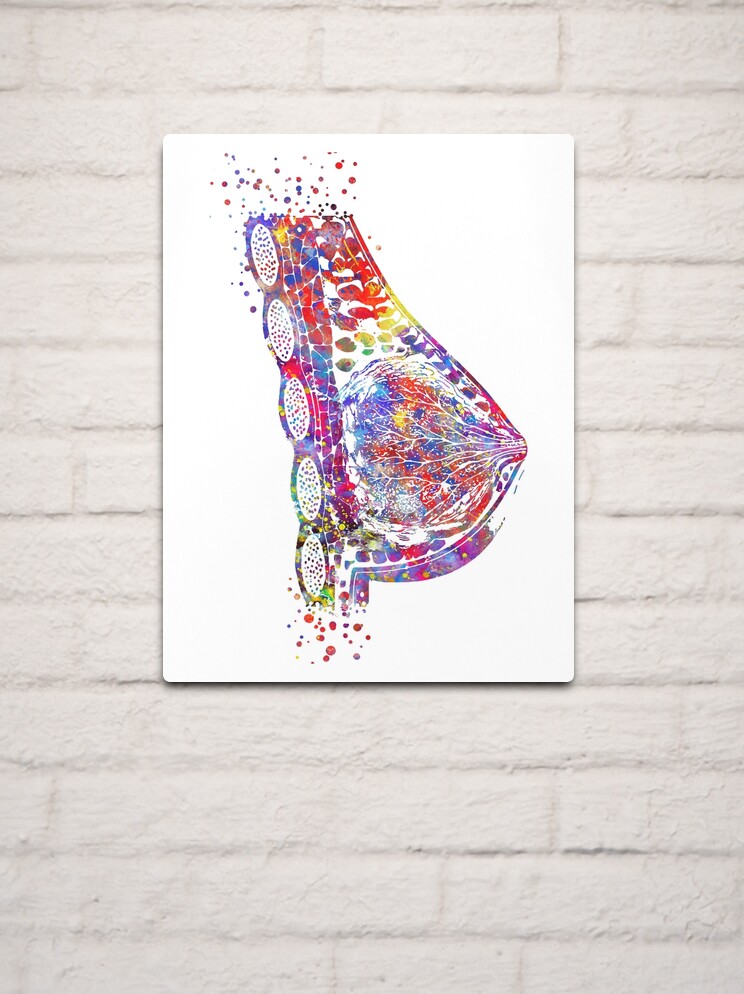A square piece of artwork is mounted on a white brick wall, serving as a striking focal point. The artwork, set against a white background, depicts an abstract, bohemian representation of a female breast in a side profile. The breast is portrayed with intricate detail, showcasing the milk ducts rendered in a vibrant array of colors. The image features a rounded triangular shape, extending to a point at the three o'clock position. Pastel shades of blue and green outline a series of five circles arranged in an almost straight line on the left. Towards the right, the triangular shape encompasses splashes of color such as red, blue, yellow, light gray, light blue, and a tweed-colored brownish-green. These hues suggest a mix of anatomical precision and artistic flair. The bottom part of the triangle curves gently, and the top and bottom edges are adorned with multicolored paint splatters, giving the impression of flicks from a paintbrush. The overall effect is a visually captivating blend of anatomical art and vivid abstraction, making it a truly unique piece that stands out against the stark white brick background.